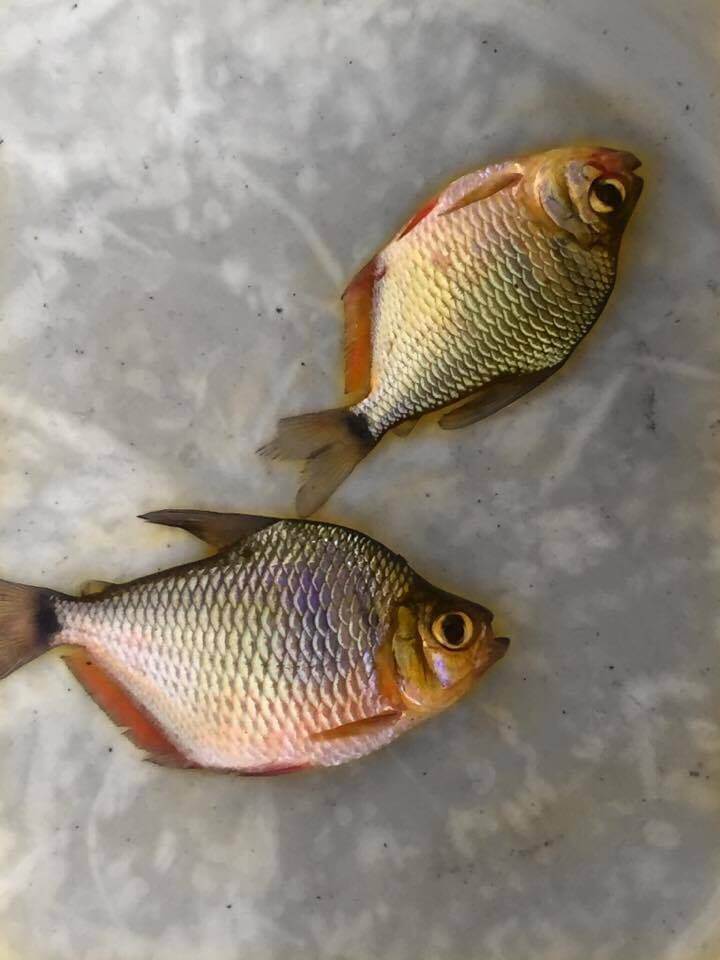The image depicts two small, recently deceased goldfish laying in the bottom of a white, stained bucket. One fish lies on its side, while the other is upside down above it. Both fish display a shiny gold tint to their bodies, covered in small, detailed scales. The fish have distinctive red fins along their bellies and brown dorsal and tail fins. Their yellow eyes, accented with large black pupils, remain wide open, and their mouths are agape. Despite the close zoom, the fish are clearly laid out with no other objects visible in the frame.